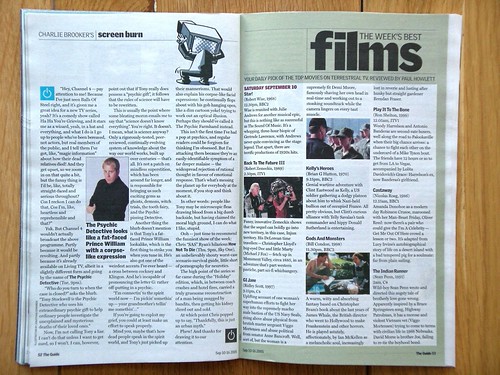In this photograph, a wooden table serves as the backdrop for an open magazine, specifically displayed on its fourth row. On the left page of the magazine, various articles can be seen. The right page features eight small, concise articles under the heading, "Films: This Week's Best," which is prominently highlighted in a khaki-green color. The subheading titles are written in red, making them stand out against the background. Additionally, on the left side of the layout, there is a distinct cartoon illustration depicting a character carrying a computer, adding a whimsical touch to the page's aesthetic.